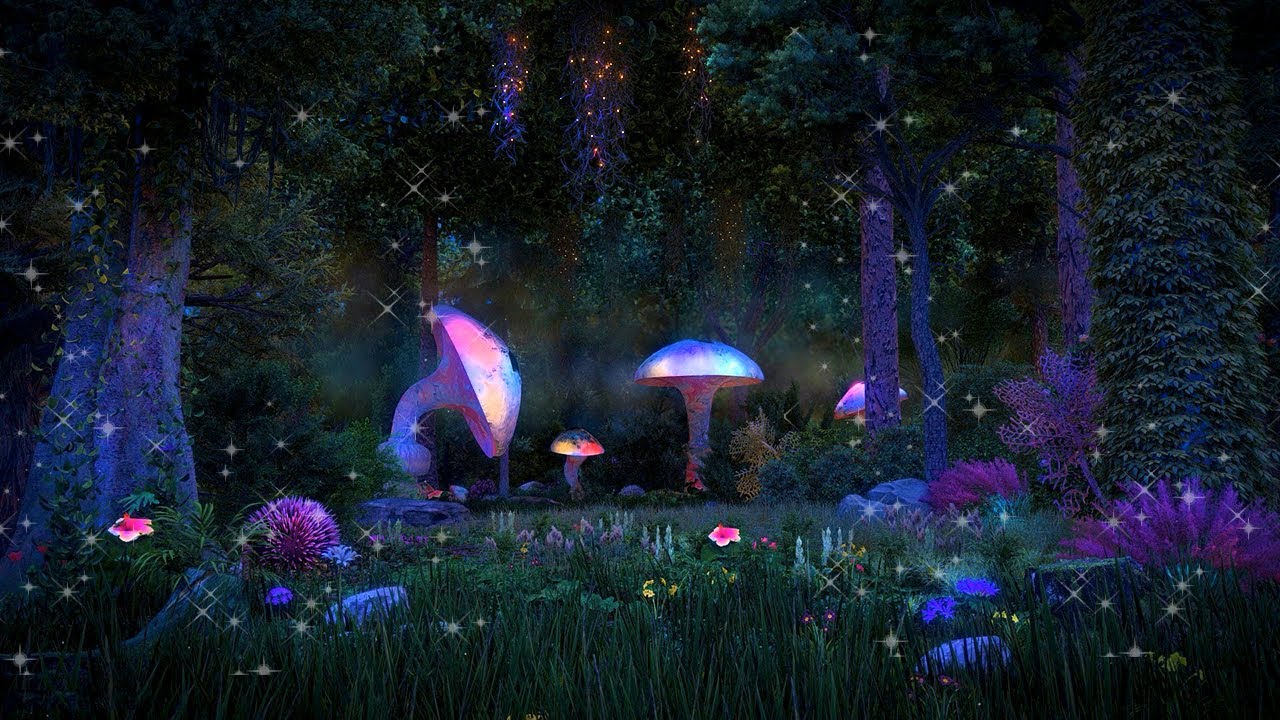In this highly detailed fantasy-themed graphic image, we observe a magical forest scene bathed in the enchanting glow of night. The image is dominated by several glowing mushrooms that emit a bright pinkish-whitish light, nestled amidst large, densely clustered trees with dark green and black foliage. These mature trees, some with bark visible and others draped in leaves, frame the scene, contributing to the mystical ambiance.

Among the trees, which are colored in shades of deep green and almost blue, there is a tree covered in leaves on its side. On the left side of the image, you can see the bark of another tree, adding texture and depth to the scene. The ground is covered in tall, vibrant green grass interspersed with bright purple plants and flowers, contributing to the lush undergrowth of this enchanted forest.

At the heart of the scene, three distinctive mushrooms stand out: one bent over to the right, a smaller one in the middle, and another mushroom next to it. These mushrooms, varying in shades of purple, green, and blue, have rounded caps that add to the magical aesthetic, especially with the light they emit.

In the air, shimmering white twinkles, reminiscent of stars, and sparkles create a whimsical atmosphere. There are also bright reddish-orange fireflies appearing mostly near the treetops, enhancing the night-time fairyland vibe. The distant background shows a star-studded sky, adding to the overall ethereal feel of this enchanted forest setting.